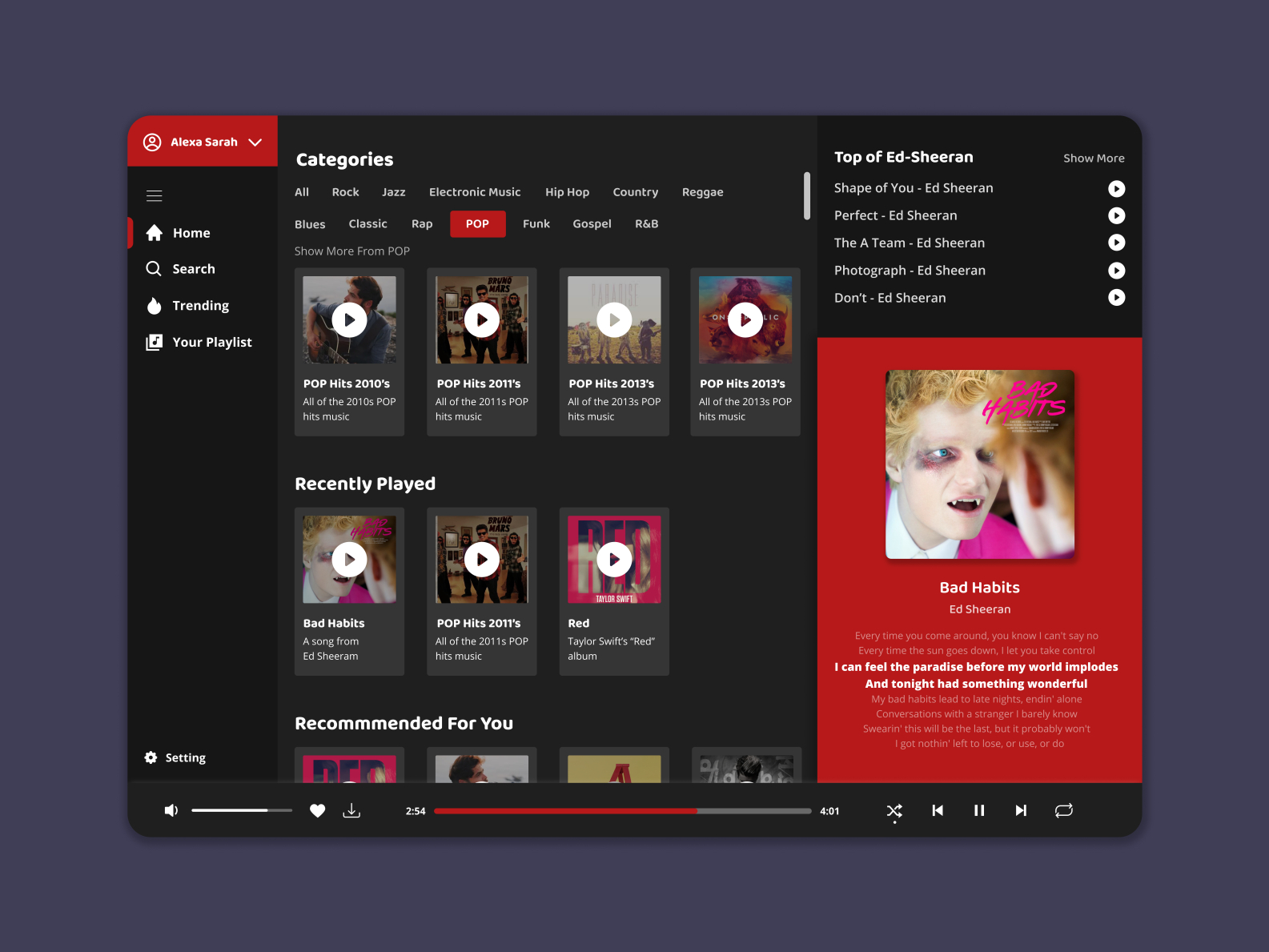A detailed and cleaned-up caption for the image could be:

---

**Music Website Interface Overview**

This image depicts the interface of an unidentified music website. In the top left corner, a red bar features a small profile image labeled "Alexa Sarah". Below the red bar, a vertical menu runs down the left-hand side of the page. The menu includes options such as Home, Search, Trending, and Your Playlist, all in white text, with the Home button highlighted by a red accent.

Adjacent to the main menu, a column lists music categories: All, Rock, Jazz, Electronic Music, Hip Hop, Country, Reggae, Blues, Classic, Rap, Pop, Funk, Gospel, and R&B. The Pop category is highlighted in red. Within this section, there is a prompt to "Show More from Pop," followed by a series of pop hits from different years: Pop Hits 2010s, Pop Hits 2011s, Pop Hits 2013s, and a repeated listing for Pop Hits 2011s.

Highlighted songs include "Bad Habits" by Ed Sheeran and "Red" from Taylor Swift's album "Red". A "Recommendations for You" section is also visible.

An image related to Ed Sheeran is displayed on the side, featuring some of his top hits such as "Shape of You," "Perfect," "A-Team," "Photograph," and "Don't." The cover art of the album "Bad Habits" is visible, accompanied by the lyrics: "I can feel paradise before my world implodes. And tonight had something wonderful."

---

This caption provides a comprehensive and structured description of the website layout and content as shown in the image.